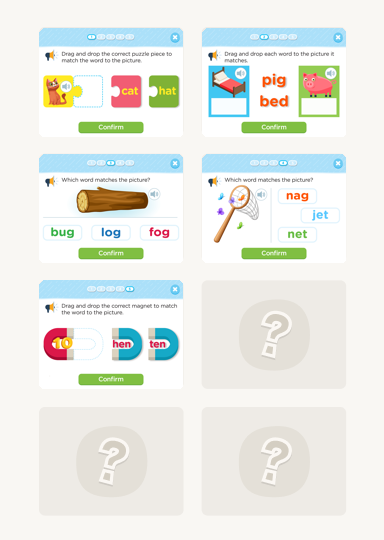In the top left corner of the image, there is a square with three puzzle pieces. The first piece, yellow, features a cat and a volume icon. Next to it is a pink piece with the word "cat," and a green piece labeled "hat." Below these pieces, the word "confirm" is displayed. 

Adjacent to this is another square displaying a bed labeled "pig in bed," with an illustration of a pig next to it and the word "confirm" below.

Below these, a square shows a wooden-handled net catching butterflies, accompanied by the words "nag, jet, net" and the word "confirm" beneath it. 

To the left of this, there is a square featuring a brown wood log with the words "bug, log, fog," followed by the word "confirm." Within the same square, there is also a red magnet labeled "10," a blue magnet labeled "hen," and another blue magnet labeled "10," all followed by the word "confirm."

To the right, there is a gray square with a lighter gray circle and a gray question mark inside it. Identical gray squares with the same content are located below and to the left of this square.

The entire background of the image is a uniform gray color.